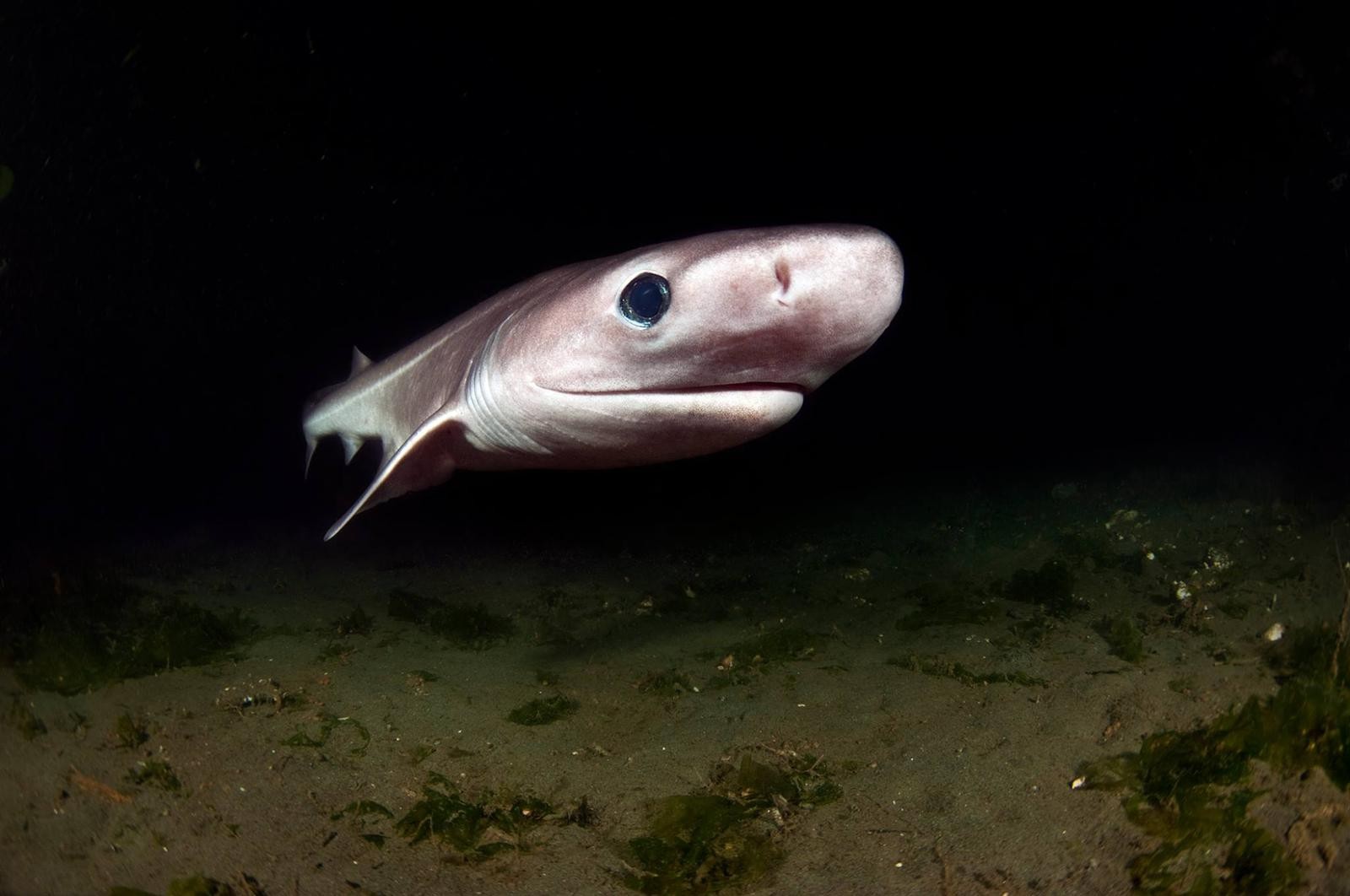This underwater photograph, likely shot in deep, dark waters, captures a silvery white to light gray bull shark swimming closely above the sandy seafloor, which is lightly illuminated by the camera's flash. The ocean bottom is a sandy light brown dotted with patches of green moss and floating kelp. The shark, estimated to be about five to six feet long, is centered in the image and shown in a side profile. Its wide nose, one large eye with a bluish tint, and the thin line of its closed mouth stretching from nose to eye are clearly visible. The background is very dark, almost black, providing a stark contrast to the illuminated seafloor and the shark’s silvery highlights near its fin and mouth, with one fin visible and the body extending all the way to the tail. This professional photograph likely taken by a scuba diver presents a detailed and striking view of the shark in its natural, deep-water habitat.